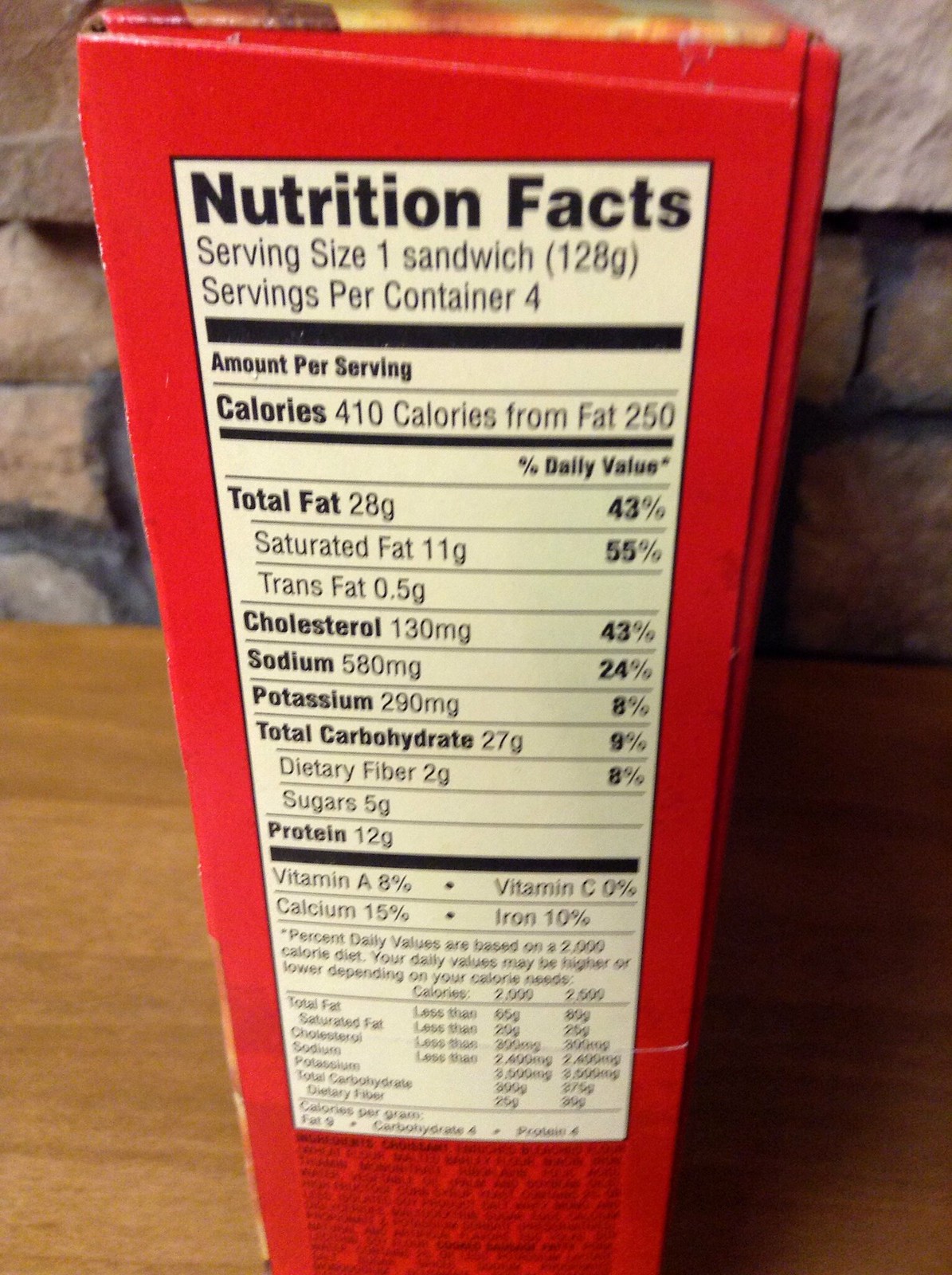The colour photograph captures a close-up of the narrow side of a food box, showcasing the Nutrition Facts label. The label, while slightly blurred and out of focus, denotes a serving size of one sandwich (128 grams) and indicates that there are four servings per container. The image suggests that the product is a pack of sandwiches. The photo is angled slightly top-down, and the upper portion of the box is cropped out of the frame. The background consists of a brick wall, adding a rustic touch to the scene. The box rests on a wooden table, with the grain visible running horizontally from left to right. The table's right side is cast in deep shadow, contrasting with the mid-brown tone of the illuminated left side.